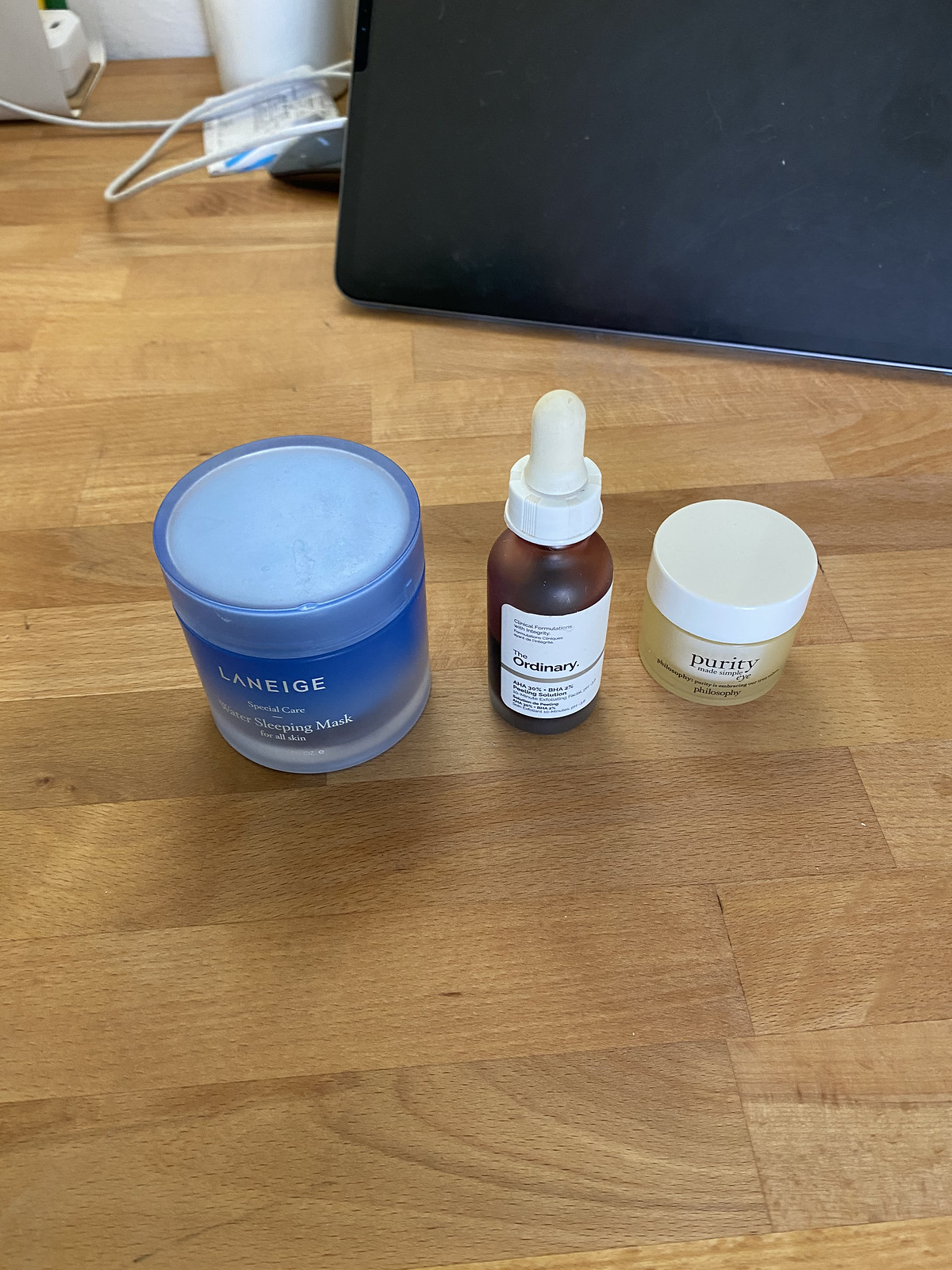This high-angle photograph features a rustic light honey-colored wood table with thin panels running horizontally, showcasing a mix of gray and brown hues that contribute to its worn, vintage charm. In the background, there is a glimpse of a wall plug with a cord extending from it, and some white objects, one cylindrical in shape, situated in the top left and back of the frame respectively. 

Dominating the upper section of the image is a partially visible computer screen with a sleek black frame, appearing to be propped up on the table with an unseen stand. 

Centrally positioned below the screen are three distinct objects: 

1. A blue container with a lid labeled "La Neige," identified as a sleeping mask.
2. A brown bottle marked "The Ordinary," featuring a white label and a dropper dispenser commonly used for serum or liquid skincare products.
3. A tan container with a white lid bearing the name "Purity."

Each item is neatly arranged, drawing attention to the varied textures and colors that provide a juxtaposition to the rustic wooden table.